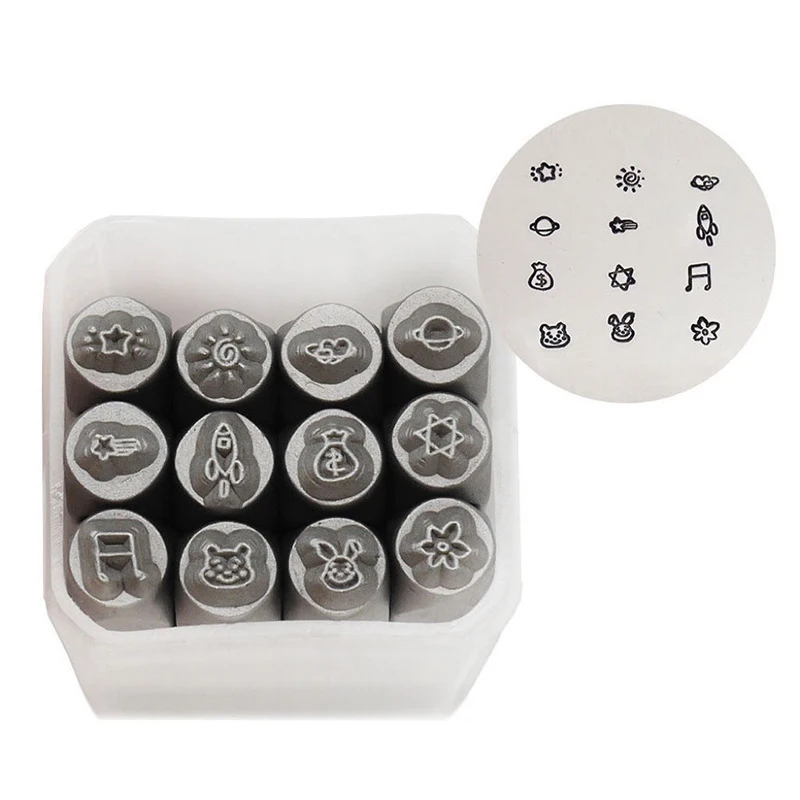This black-and-white photograph showcases a neatly arranged box containing 12 circular rubber stamps, each adorned with a distinct graphic. The box, with its rounded edges and measuring approximately 12 inches in all dimensions, features symbols such as a spaceship, a money bag, a rabbit face, a bear face, a six-pointed star (possibly the Star of David), a planet with a ring (likely representing Saturn), a swirl, two hearts, a star with a streak, a flower, a music note, and a pig. Positioned to the right of the box is a smaller, circular graphic that serves as a reference chart, displaying stamped impressions of each graphic found in the box. This detailed chart aids in visualizing the designs these stamps create when inked and pressed onto paper, hinting at their potential use for art projects or catalog demonstrations. The image is devoid of any background elements, emphasizing the stamps and their designs, and was likely cropped for a catalog presentation.